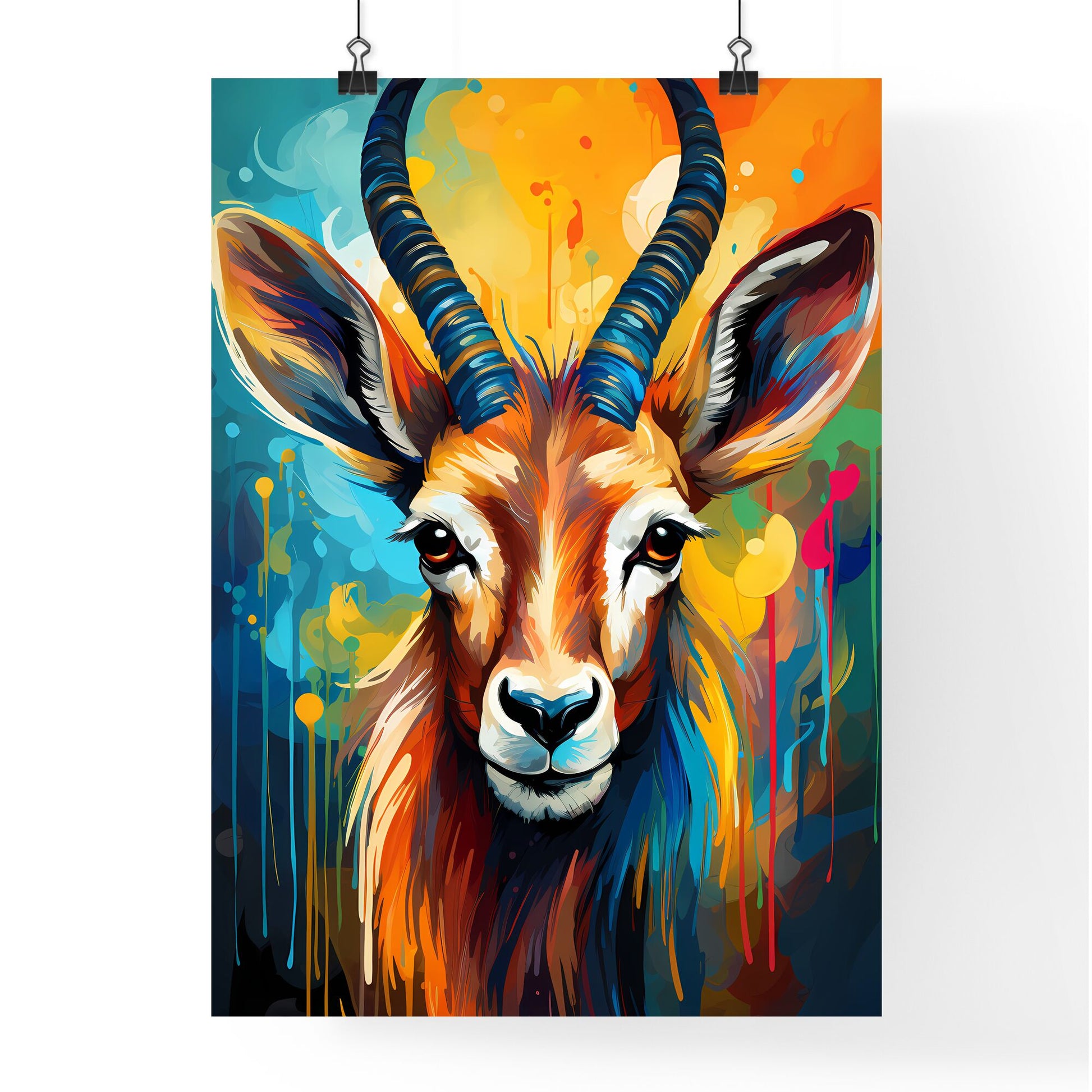This is a striking and vibrant painting of a horned deer, rendered with a surreal, kaleidoscopic array of colors. The image captures the deer's head facing forward, with two blue horns featuring occasional brown stripes that rise elegantly above and curl slightly. Vibrant yellows, oranges, and blues dominate the background, blending in a dynamic, dripping paint style that adds a sense of movement to the piece. The deer's ears stand tall, colored with black, blue, and white. Around the deer's expressive brown eyes and muzzle, there are areas of white, contrasting with its predominantly brown coat. The deer’s nose is brown, and a strip of white fur runs down the middle of its nose. Underneath the chin, there is a mane-like texture that transitions from the natural browns and whites of the fur to an array of blues, yellows, and hints of red. The entire image is a visual feast of colors and dripping effects, creating a surreal and mesmerizing work of art.